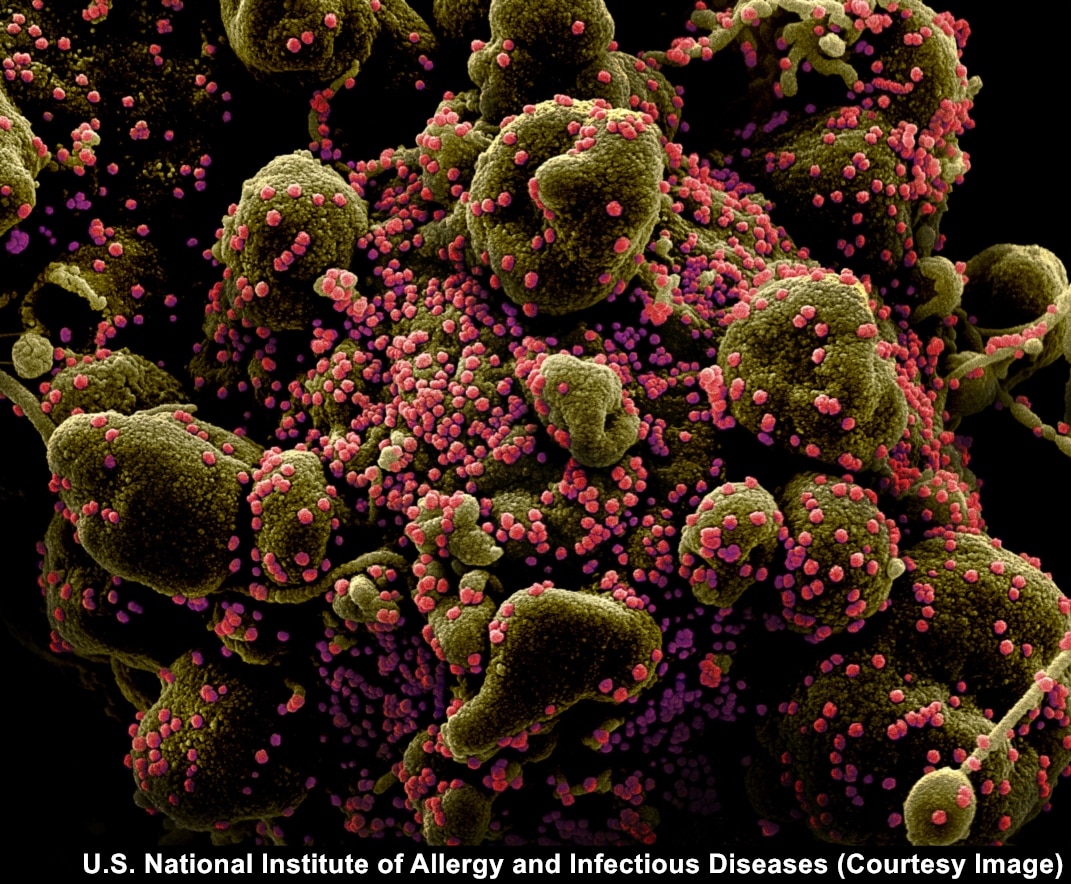This highly detailed microscopic image, courtesy of the U.S. National Institute of Allergy and Infectious Diseases, reveals an intricate, close-up view of a green, organic surface covered in bulbous, bumpy structures. Each of these uneven green blobs is adorned with numerous tiny, circular pink spores, giving the appearance of a virus or bacterial colony spreading across the surface. The texture resembles reptilian scales interspersed with pink growths. The whole structure protrudes in a circular shape with multiple extrusions against a stark black background, making the brightly colored organic mass stand out vividly.